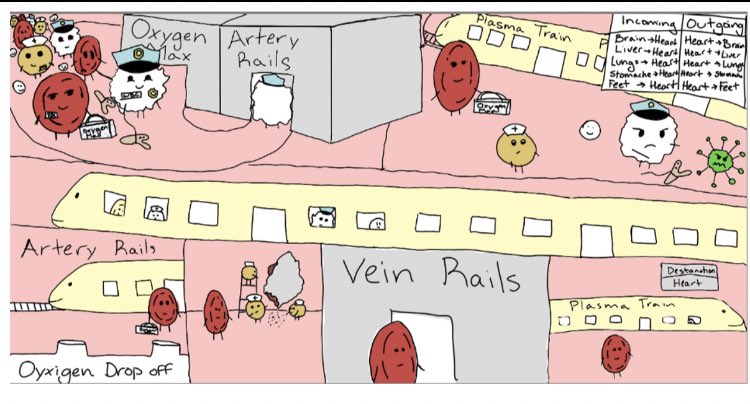This intricate illustration resembles a comic strip and serves as a detailed diagram of the circulatory system. In the center is a vibrant, yellow horizontal strip representing the plasma train, with windows showing various cells looking out. Above, boxes labeled "Oxygen Max" and "Artery Rails" depict red and white blood cells preparing to enter a building for oxygenation. The artery rails guide them, dotted with blood droplets, toward the oxygen drop-off point. Detailed captions throughout indicate the paths: "Incoming," "Outgoing," "Brain to Heart," "Feet to Heart," and more, clearly mapping the circulatory journey. One red blood cell disembarks at the oxygen drop-off, then rejoins the vein rails for the return trip to the heart. A white blood cell is shown combating a green bacterium below, underscoring the body’s defense mechanisms. The right side features another plasma train, a legend signifying various destinations like the brain, heart, and lungs, and a corner labeled "Destination Heart." The bottom part has the vein rails and plasma train departing with the heart symbol indicating the central hub of circulation. Each element, including a yellow sphere with a nurse's hat, serves to educate viewers on the circulatory process, making the complex system accessible and engaging.